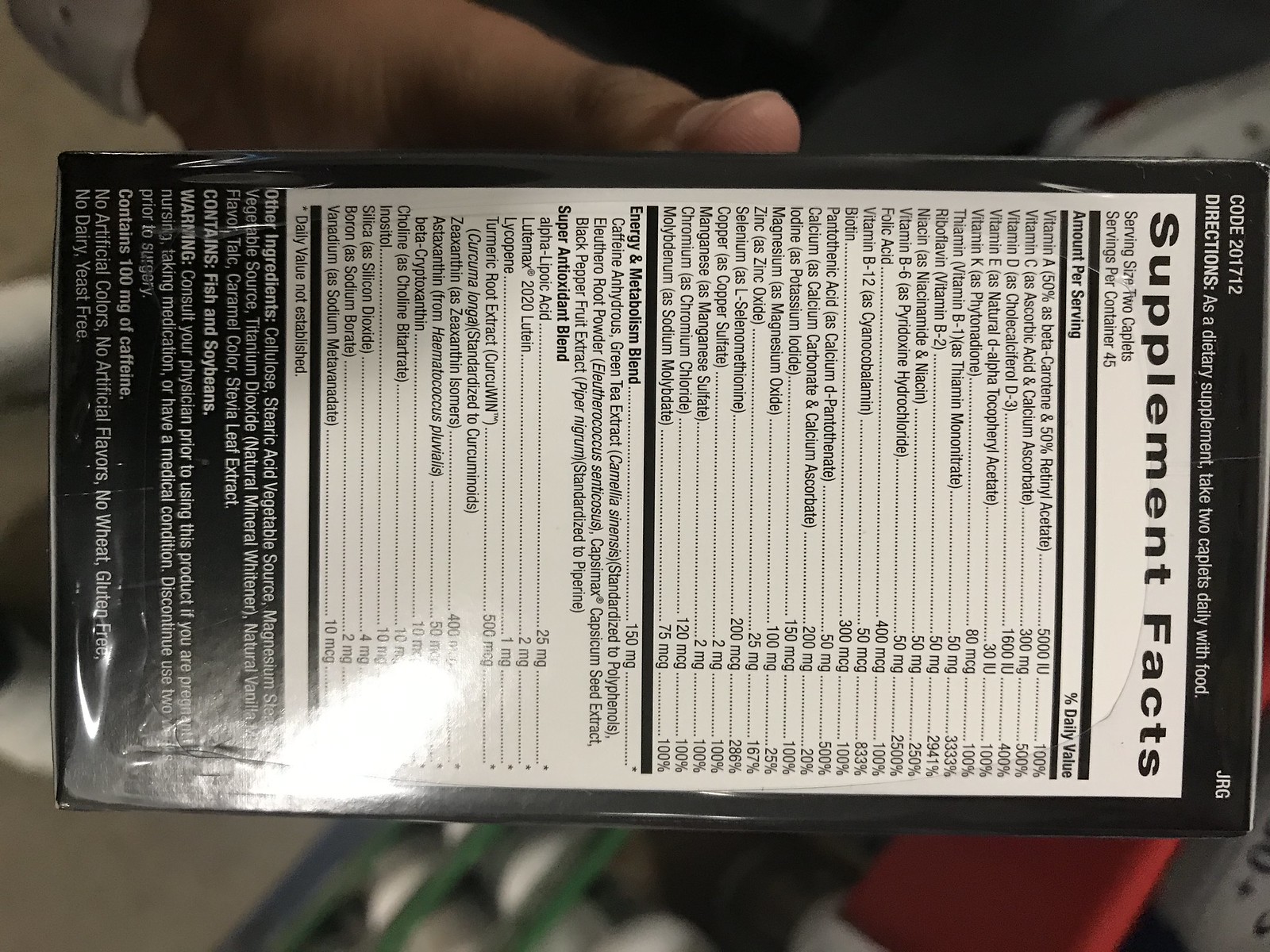The photograph captures a person holding a black dietary supplement box sideways, making it slightly challenging to read. The image focuses on the supplement fact sheet on the box, which is presented within a white rectangular area. This sheet details an extensive list of nutrients, including vitamins A, C, D, E, and K, as well as B-complex vitamins such as thiamine, riboflavin, niacin, B6, B12, folic acid, biotin, and pantothenic acid. It also lists various minerals like calcium, iodine, magnesium, zinc, selenium, copper, chromium, molybdenum, boron, and vanadium. Additionally, the sheet mentions an energy and metabolism blend featuring ingredients such as caffeine, green tea extract, ethyl root powder, capsicum seed extract, and black pepper fruit extract. Other components include superoxide blend, alpha-lipoic acid, lutemax, liposine, turmeric root extract, zeaxanthin, astaxanthin, beta-carotene, choline, inositol, and silica. The product boasts no artificial colors or flavors, is gluten-free, dairy-free, and yeast-free. Although there's a flash causing some glare, making parts difficult to read, the comprehensive nutritional information and specifications of serving size—two caplets per serving with 45 servings per container—are clearly visible.